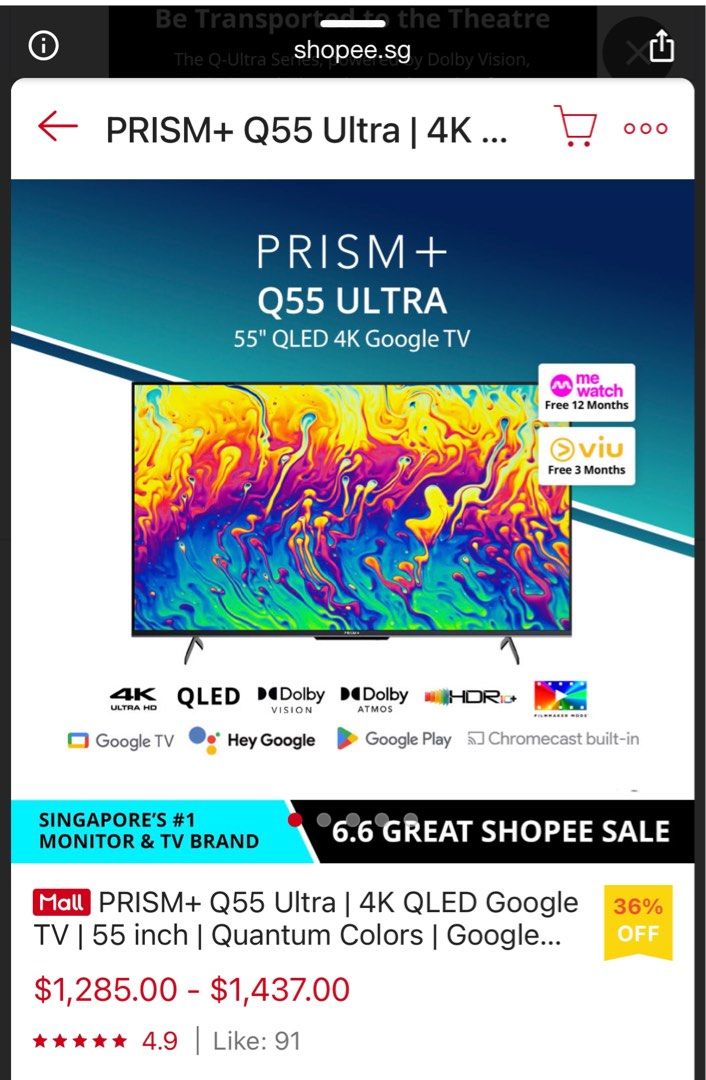This is a detailed screenshot likely taken on a phone or tablet. The background features an open window displaying the message "Be transported to the theater." In the foreground, the main focus is on a detailed advertisement for a Prism Plus Q55 Ultra 4K TV, suggesting that the user has selected this specific model to view more information.

At the top of the forefront window, there's a white strip with a left-pointing red arrow on the left. To the right of the arrow, the text "Prism Plus Q55 Ultra 4K" is written in black. Below this, there's a red card icon and three red dots.

The main section of the image showcases the TV model "Prism Plus Q55 Ultra" in bold white text against a bluish gradient background. The TV screen displays a vibrant, colorful abstract design reminiscent of flowing oil, featuring an array of colors including yellow, orange, red, purple, dark blue, light blue, greenish-blue, neon green, and more.

To the right of the display, promotional details are highlighted: customers receive a Mi Watch free for 12 months and VIU free for 3 months with the purchase of the TV. Additionally, the TV boasts features like 4K Ultra HD, QLED, Dolby Vision, Dolby Atmos, HDR, Google TV, Hey Google, Google Play, and Chromecast built-in.

The advertisement emphasizes that this model comes from Singapore's number one monitor and TV brand and is part of the "6.6 Great Shopee Sale," currently offering a 36% discount. The TV price ranges between $1,285 and $1,437. It has an impressive rating of 4.9 out of 5 stars and has been liked 91 times.